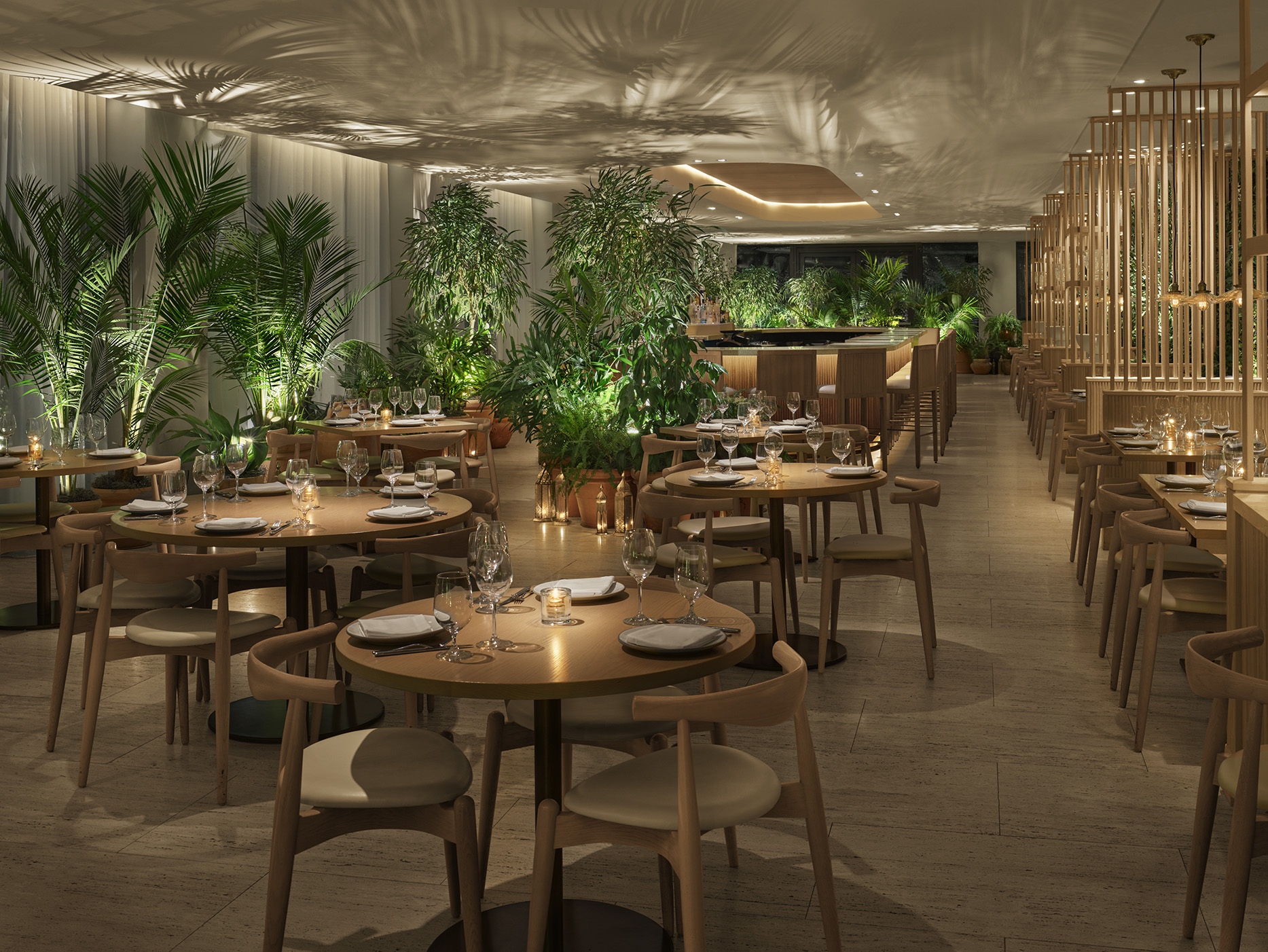The photo showcases an elegantly set empty restaurant, ready to welcome its guests. The tables, mostly wooden and circular, are dressed with plates, napkins, silverware, and glasses of wine, giving an air of sophistication. The restaurant's color scheme is dominated by shades of beige, accentuating its classy ambience. Large potted plants and vibrant greenery add splashes of green throughout the space, with shadows from the greenery projected onto the ceiling by the strategically placed lighting. In the background, a bar area is situated, providing a focal point amidst the lush decor, and some booths are separated by golden fencing, enhancing the restaurant's refined interior. The overall design, with its mixture of nature and elegance, creates a welcoming and upscale atmosphere.